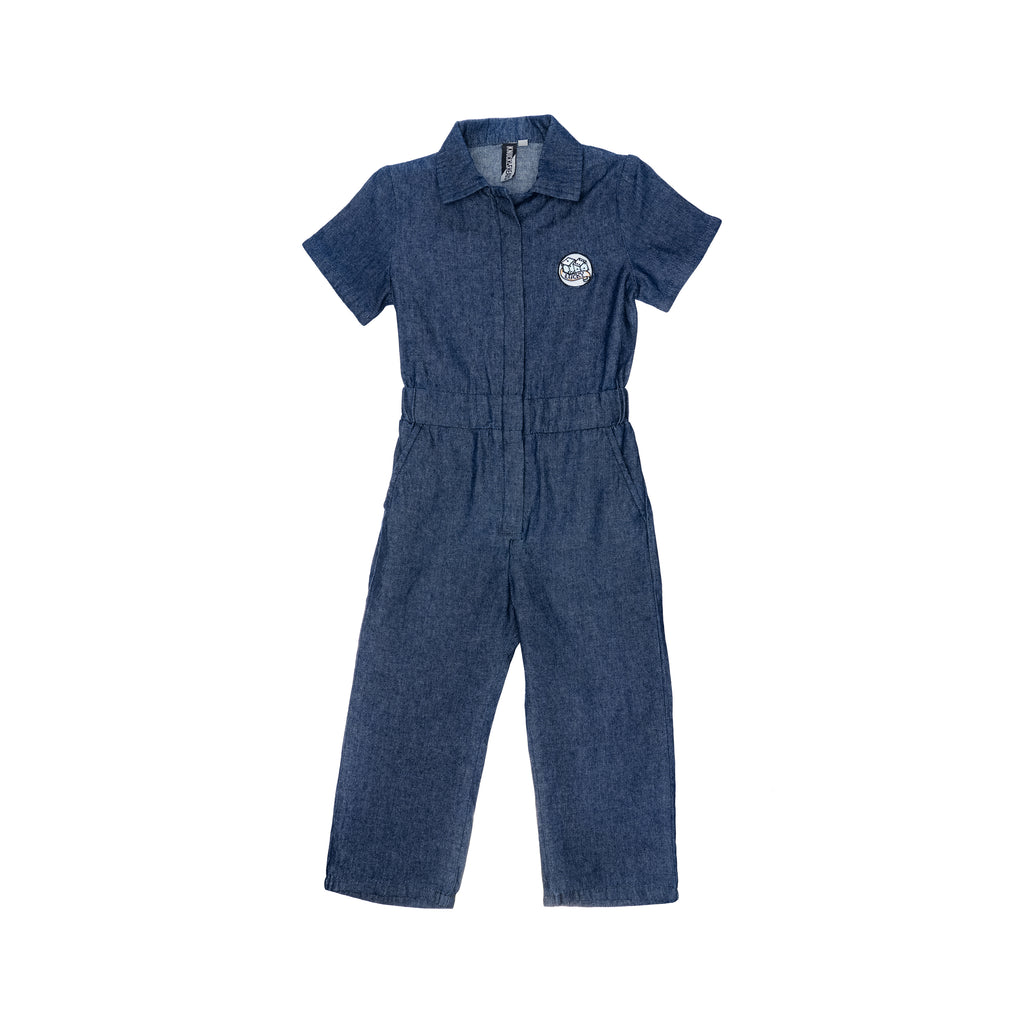This image showcases a blue, casual one-piece jumpsuit set against a white background. The jumpsuit appears to be made of denim material and features short sleeves and a collared, button-up top. It has a cinched waist, giving it a belted appearance, and the legs extend to either below the knee or all the way to the ankle. On the left chest, there's a prominent white circular patch with an emblem displaying two dice and the word “Lucky” beneath them. Additional details include a tag with black and white rectangular detailing at the back neck area of the jumpsuit.